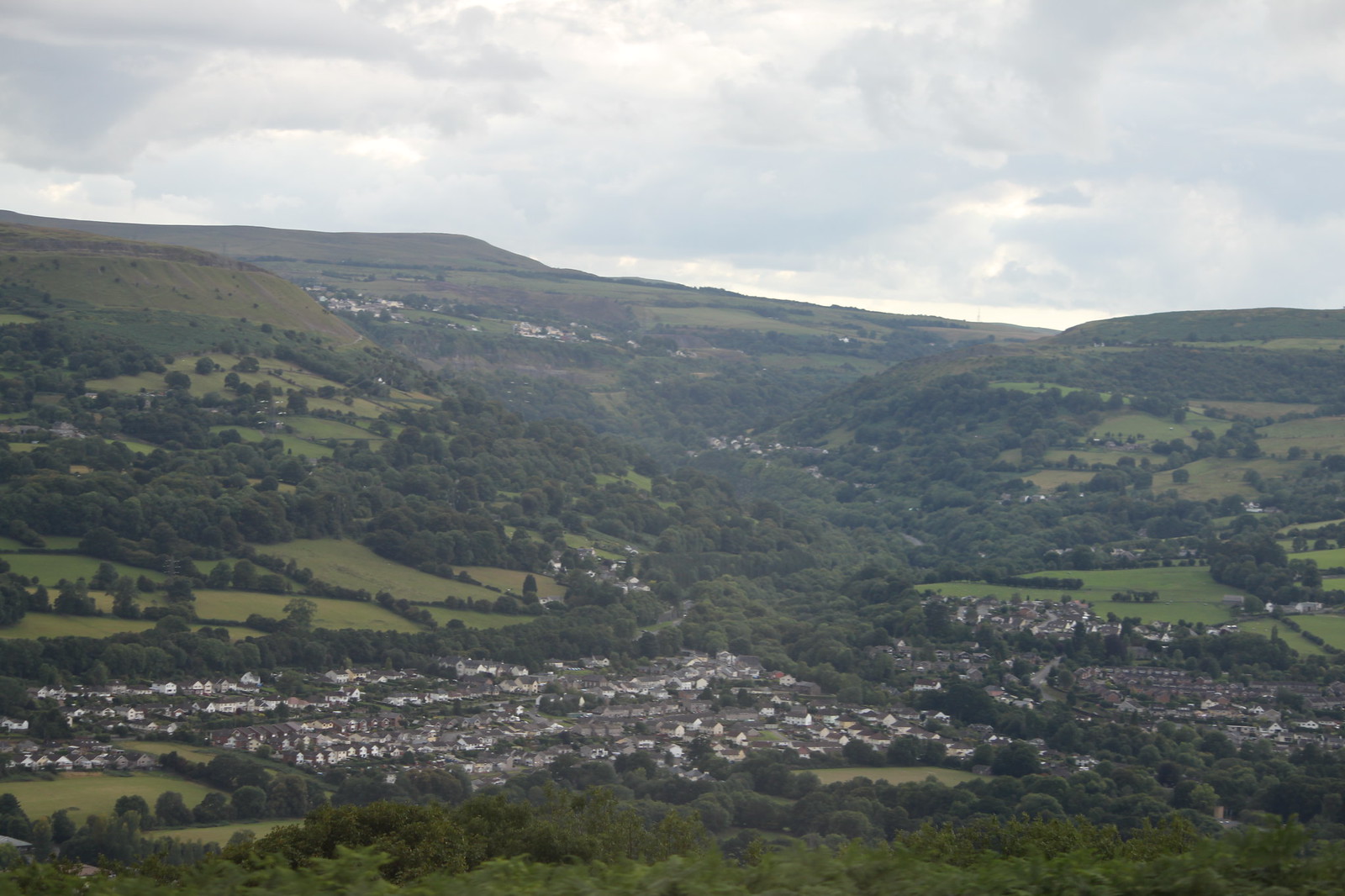This detailed aerial photograph captures the serene landscape of a small town nestled in a shallow valley, likely in Ireland or Scotland, given the distinct feel of the landscape. The town is predominantly composed of white buildings with gray roofs, clustered together and surrounded by lush greenery. Open patches of green farmland, forming square and rectangular pastures, are accentuated by rolling hills that stretch into the distance. These pastures, usually reserved for sheep, hint at the region's agricultural practices. The scenery is predominantly green, with abundant trees and grassy fields. A hazy, overcast sky with diffused clouds casts a gentle light over the landscape, creating a peaceful and tranquil atmosphere. Despite the visibility of the town's structures, the focus of the image remains on the verdant landscape, devoid of any visible people, cars, or animals, emphasizing the natural beauty of the area.